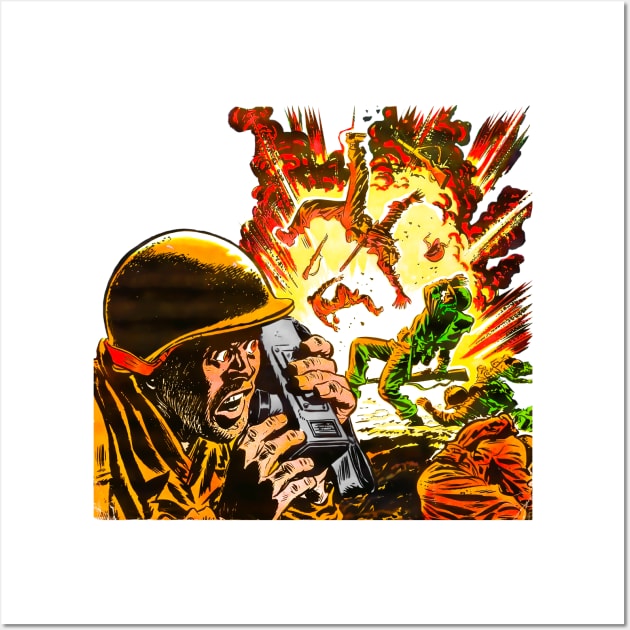The comic book-style image captures a chaotic and intense battle scene dominated by a massive explosion in the background. In the foreground, a terrified soldier with a rugged, unshaven face screams into a black walkie-talkie, his brown helmet and uniform contrasting with the vibrant orange neckband and the red trim on his helmet. Behind him, the explosion blasts several soldiers into the air, their bodies twisted violently by the force. One soldier is seen recoiling from the explosion, another one is lying down, protecting his head, while two others somersault through the air, one losing his hand and gun in the blast. The fiery hues of yellow and red from the explosion illuminate parts of the soldiers' uniforms in shades of green, emphasizing the chaotic energy of the scene. The image is devoid of text, relying on its dramatic visuals to convey the turmoil of the battlefield.